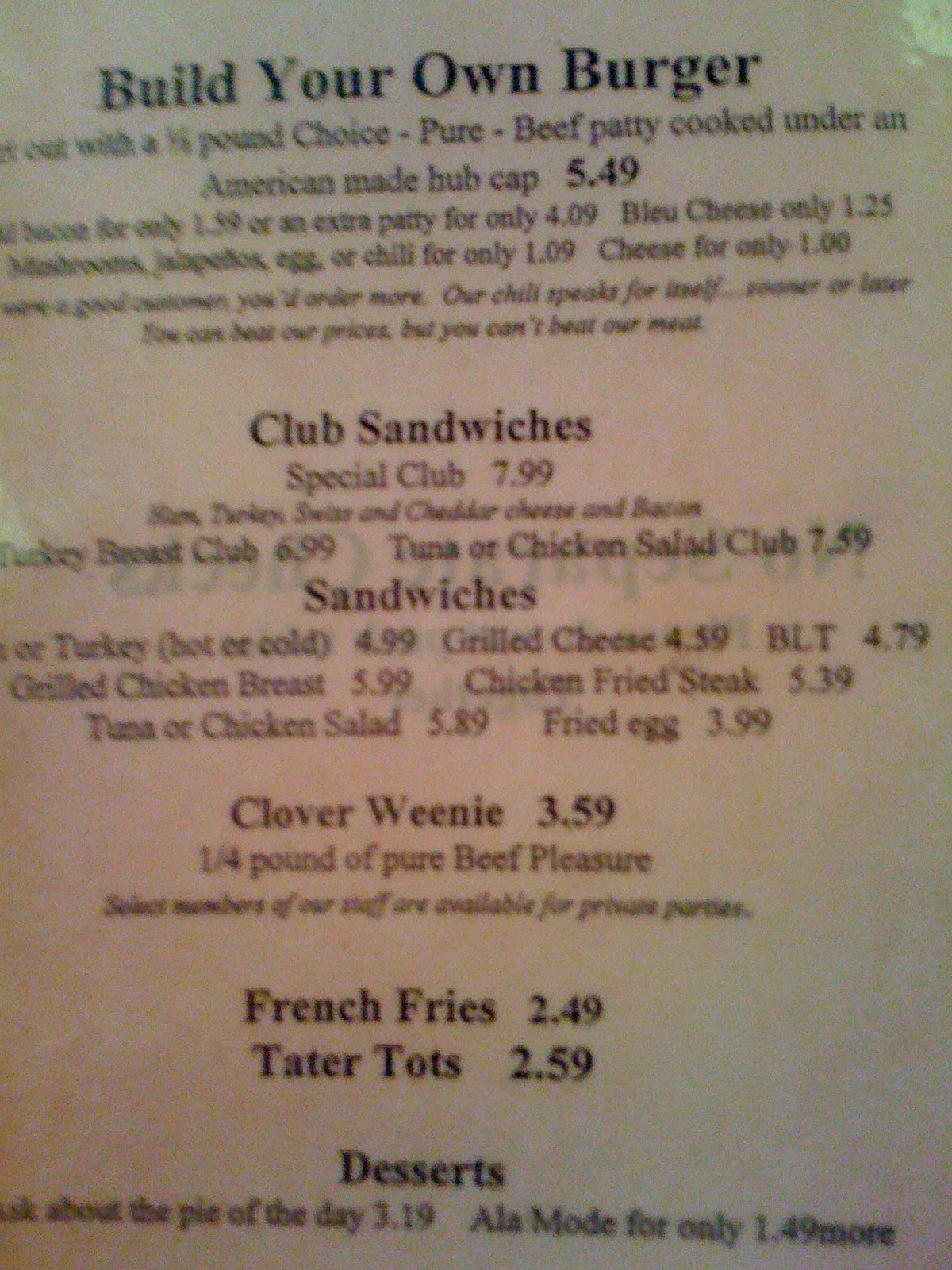This detailed photograph captures a restaurant menu with a sleek, white, glossy finish. At the top, the menu features a bold, black heading that reads, "Build Your Own Burger." This section outlines the option to choose a beef patty priced at $5.49, with a variety of additional toppings available such as blue cheese, mushrooms, jalapeños, eggs, and chili.

Following this, the menu introduces the "Club Sandwiches" category. Here, the "Special Club" is priced at $7.99 and offers toppings like Swiss cheese, cheddar cheese, and bacon. Other choices include the "Turkey Breast Club" for $6.99, and the "Tuna or Chicken Salad Club" for $7.59.

The subsequent section lists a variety of sandwiches. Options include:
- Turkey (hot or cold) for $4.99
- Grilled chicken breast for $5.99
- Tuna or chicken salad for $5.89
- Fried egg for $3.99
- Chicken fried steak for $5.39
- Grilled cheese for $4.59
- BLT for $4.79

Also featured is a unique menu item called the “Cloverlini,” priced at $3.59, described as "1 1/4 pound of pure beef pleasure."

For sides, the menu offers:
- French fries for $2.49
- Tater tots for $2.59

Lastly, the dessert section encourages diners to inquire about the "Pie of the Day," priced at $3.19, with the option to add a la mode for an additional $1.49.